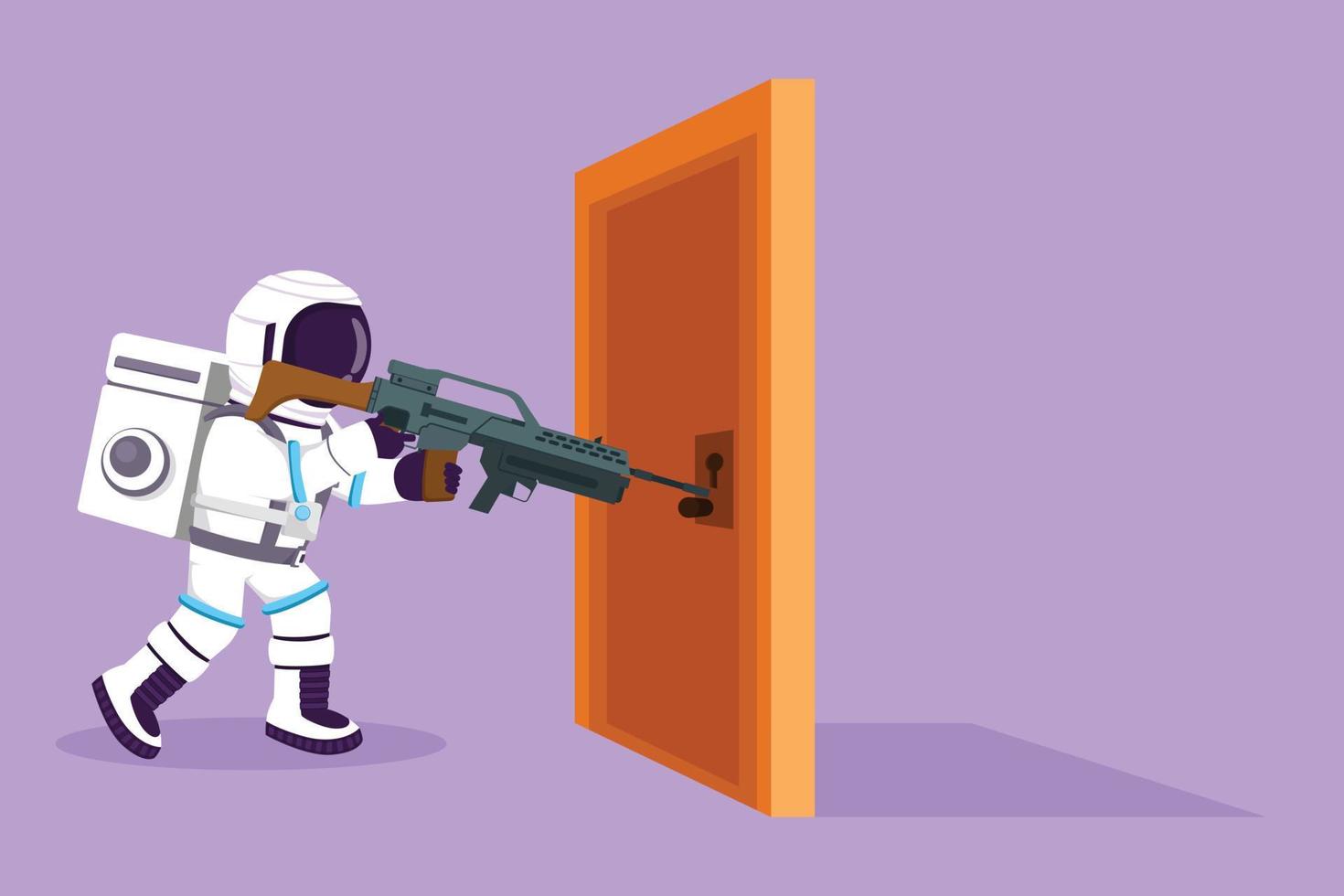This digital image showcases a detailed, computer-generated graphic of an astronaut-like figure clad in an elaborate spacesuit. The suit features distinct elements, including white pants tucked into white and black boots with blue stripes around the legs, black gloves, and a long-sleeved white jacket. Completing the outfit, a white helmet obscures the figure's face in black. Additionally, a rectangular tank, adorned with a circular detail and secured with visible buckles, is strapped to the astronaut's back. The figure is holding a semi-automatic rifle, which features a wood barrel and an elongated gray component, aimed directly at the doorknob of a bright orange door. The door fascinates with its gradient tones, darker on the inside and lighter on the outside, and peculiarly stands alone in the middle of the scene, unconnected to any structure. Behind the door, a shadow in a darker purple hue adds depth to the predominantly light lavender and purple backdrop. Positioned on the left side of the frame, the astronaut's intent gaze is fixed on the door's handle, creating a mysterious and surreal atmosphere.